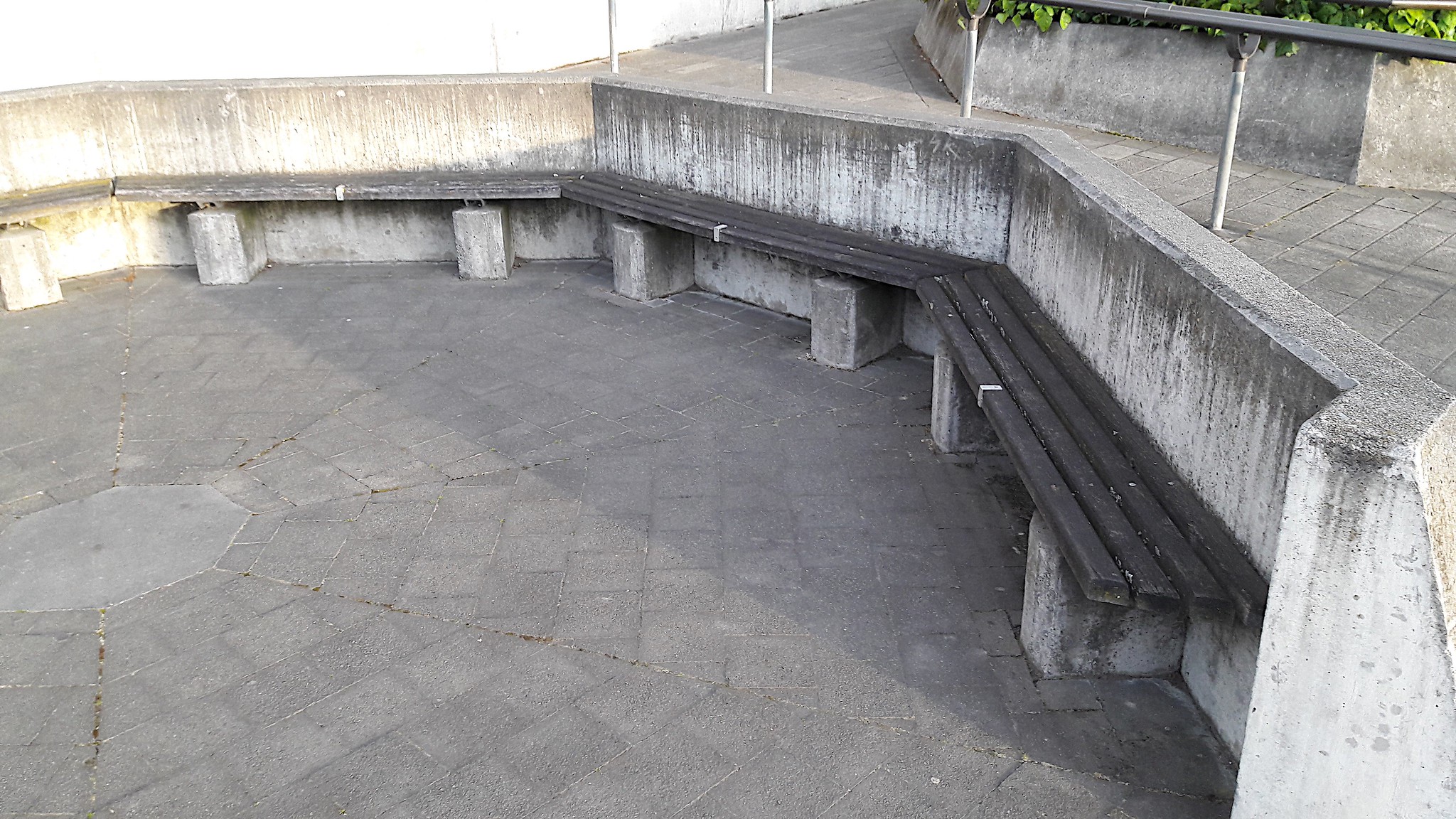The photograph depicts a somewhat grim, urban park characterized by extensive hardscaping. Central to the scene is an octagonal area paved with grey concrete tiles, possibly featuring a drain tile in the middle. Surrounding this central tile, there are multiple brick-like paver stones forming rings. Encircling the perimeter is a low, octagonal concrete wall, heavily stained and blackened by algae.

Integrated into this wall are benches built from thick concrete pillar feet supporting four wooden slats, intended for seating without backrests. These benches line the octagonal configuration of the park. Sparse greenery is visible, including small trees with protective white sleeves around their trunks, planted in openings within the hardscape, along with some plants poking through in the top right corner of the image. A black handrail with silver supports is also seen along the edge of the space. The overall feeling of the park is industrial and uninviting, with minimal landscaping amid the dominant concrete structures.